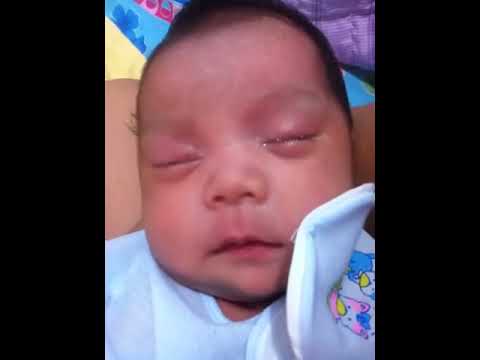The photo captures a peacefully sleeping newborn with dark black hair and very puffy eyes and face, including a slightly crusty left eye. The eyelids are noticeably puffy. The baby is dressed in a white top, possibly a onesie or pajamas, and a bib that features two kittens on the left side near the face. In the background, there are blankets with various colors and patterns, including purplish, yellow, and blue elements. Someone’s arm, likely a parent’s, is cradling the baby’s head in their elbow, providing gentle support. The image is vertically oriented, expanding beyond the frame of the letterbox view.